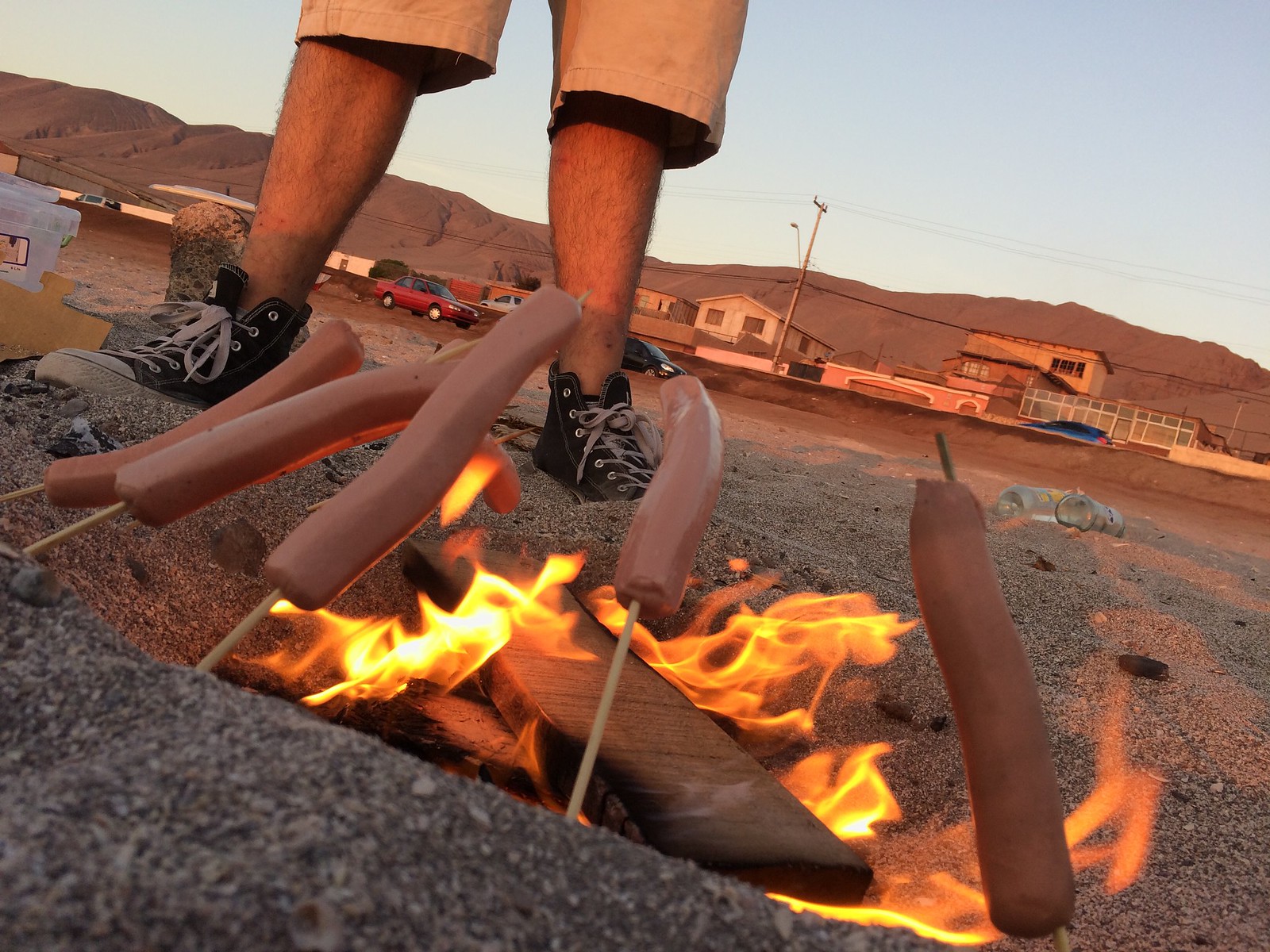The photograph captures a campfire scene set against the backdrop of a sunset, likely in a coastal or mountainous region. The image is taken from ground level, providing a close-up view of hot dogs impaled on sticks and stuck into the granulated, black and gray sandy soil, with hints of red. The fire, composed of a bunch of leaves and a few logs, is alight with yellow and orange flickering flames, roasting at least five hot dogs that are slightly glossy and not yet charred.

In the top left of the photo, a man stands with his feet clad in black high top Chuck Taylors and his knees covered by tan-colored shorts. His bare legs are visible above the sand. Beyond the man, the scene includes a red car and old-looking buildings set against reddish-brown mountains devoid of foliage. The sky is a light blue, accentuating the orange glow of the setting sun on the buildings and terrain. Two cans of some liquid are noticeable in the background, positioned on the right side behind the man.